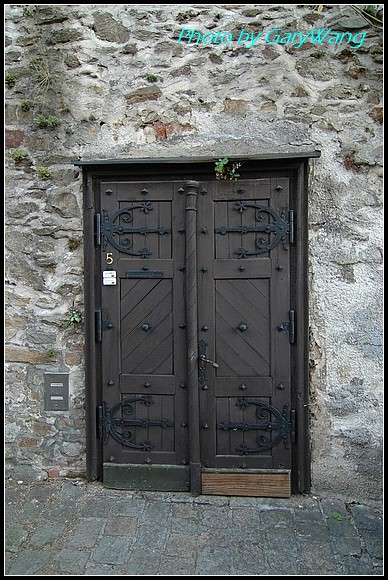This color photograph, oriented in portrait style, captures a very old, rustic front door embedded in a stone building with an irregular cobblestone construction. At the top of the image, in teal blue text, it reads "photo by Gary Wang." The centerpiece of the photograph is a wide, two-section metal door with a wooden frame. The darker wood of the door contrasts with the lighter wood planks at the bottom of both sections. The door on the right features an aged handle, while the entire door showcases numerous round, bolt-like knobs. The door's rustic charm is enhanced by black appliqué detailing on the top and bottom, resembling a half-cylinder with a line going through it, placed sidewise. The left portion of the door prominently displays the number five, below which lies a small, unreadable gold placard. The setting hints at a European ambiance, with cobblestone paving in the foreground, reinforcing the aged, historical feel of the image.